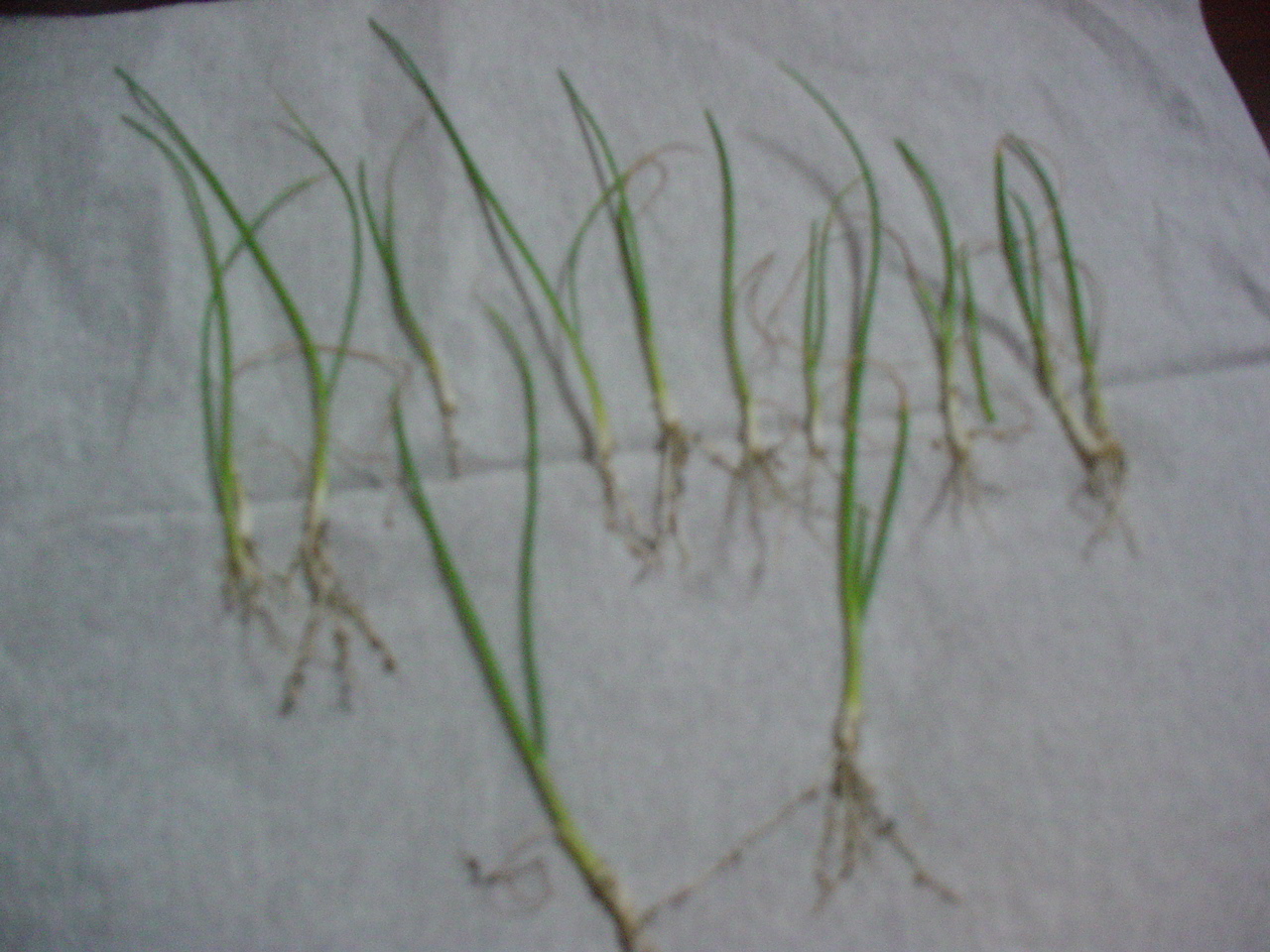The color photograph, in landscape orientation, depicts approximately ten harvested green onions arranged on a slightly creased white cloth. The onions are lined up diagonally from the top left to the bottom right. Each green onion features vibrant green leaves at the top, with the roots appearing stringy and brown, often with small clumps of dirt adhering to them. The roots fan out beneath the plants, shorter than the leafy sprout above. Two larger green onions near the bottom stand out due to their size and more prominent root structures. The photographic style is representational realism, although the image is slightly out of focus.